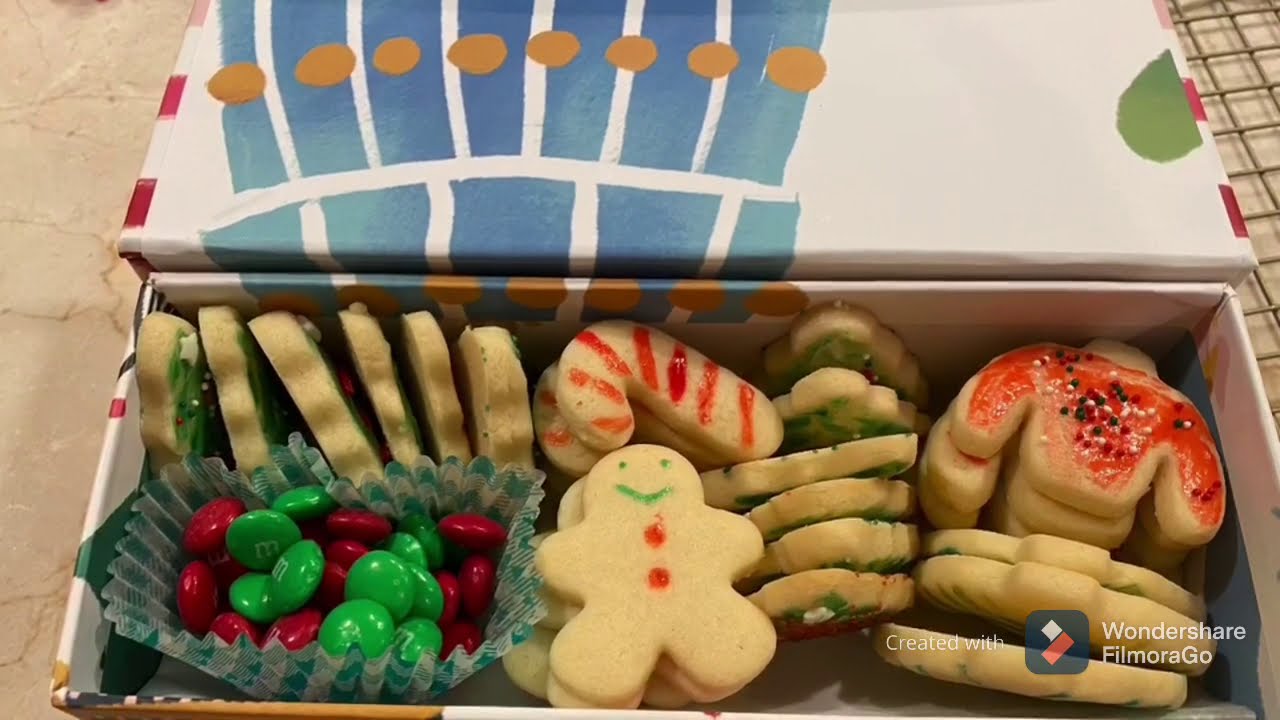The image depicts a festive rectangular tray, resembling a shoe box, overflowing with a variety of vividly decorated Christmas sugar cookies. Centered within the box is a charming gingerbread man cookie, adorned with green eyes, a green line for a mouth, and two red buttons. Above this cookie, a yellow candy cane cookie with red stripes stands out. To the left, cookies shaped like Christmas trees are visible, adorned with green icing and white stars, stacked in neat rows. A small bag of red and green M&M's nestles in a cupcake liner at the box's bottom-left corner. On the right side of the box, cookies shaped like jackets appear, with red icing and black and white sprinkles. The box itself, primarily white with blue and gold dot decals, features a logo and the text "Created With Wondershare Filmora Go" at the very bottom. Another closed box behind the tray features a contrasting design with blue squares, white lines, and a green thumbprint on the right side.